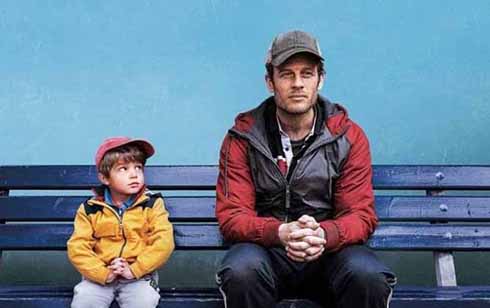In this full-color, horizontally-aligned rectangular photograph, likely from the early 80s, a man and a young boy are seated on a painted navy blue wooden bench, set against a matching blue wall. The adult male, who has short brown hair partially concealed by a gray baseball cap, wears a red and gray jacket over a partially open polo or button shirt, black pants, and black-and-white striped jogger-style pants. He sits with a serious expression, hands clasped in front of him, looking straight ahead. Beside him, the young boy, around 4 or 5 years old, glances up at the man. The boy is adorned in a red baseball cap, a yellow jacket with black accents, a blue polo shirt, and gray or khaki pants. Both subjects have their hands folded and exhibit short brown hair, contributing to a cohesive visual symmetry. The overall composition, with its color-coordinated elements, conveys a sense of stillness and introspection.